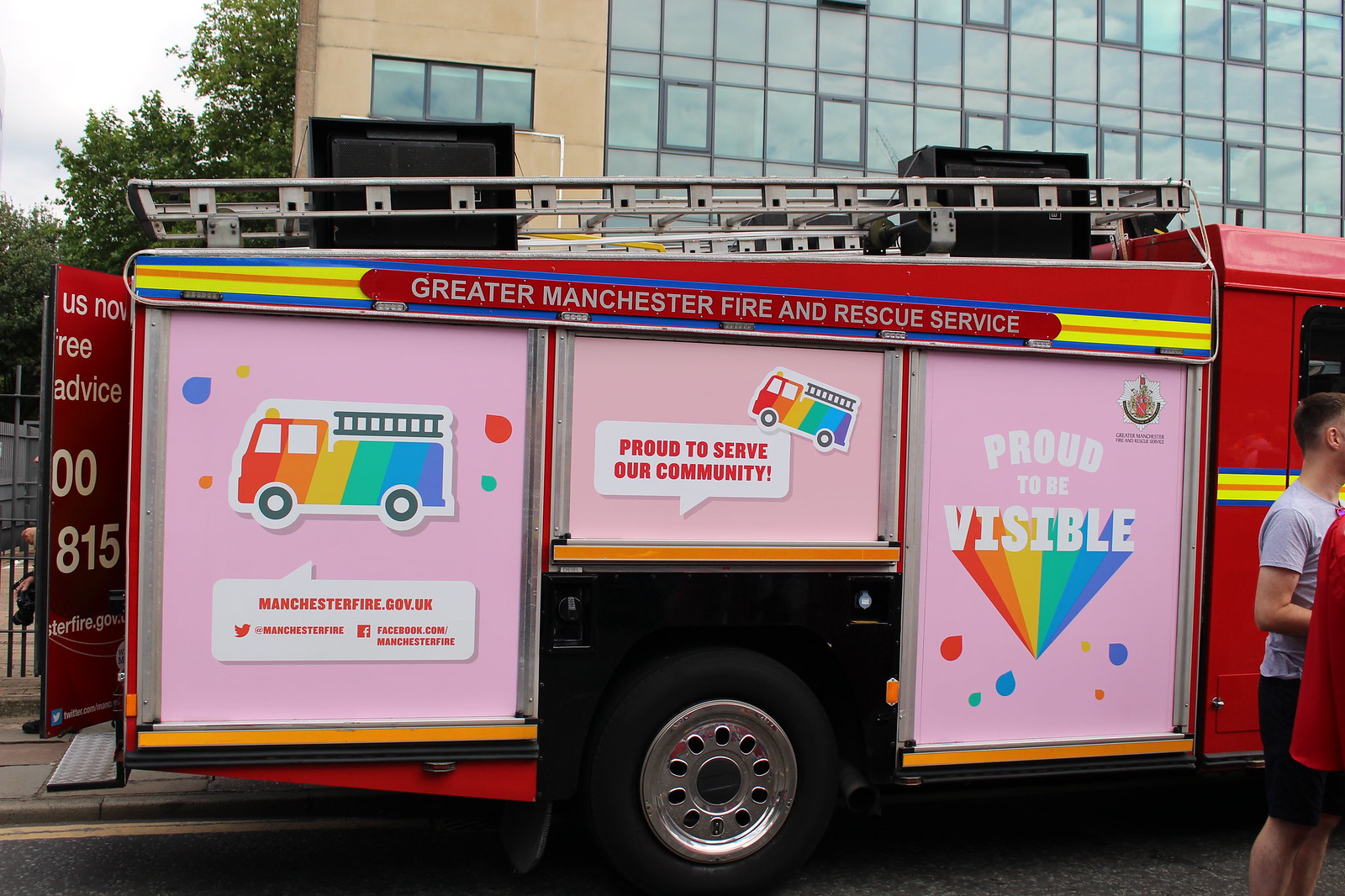This horizontally aligned, landscape-oriented color photograph features a detailed view of the side of a decorated fire truck from the Greater Manchester Fire and Rescue Service. The backdrop consists of a multi-level brownstone building with a facade dominated by rectangular windows, and in the upper left corner, the gray and cloudy sky peeks through, adorned by the silhouettes of trees behind the building.

Dominating the foreground is the side of the fire truck, displaying back doors that are open and ladders mounted on top. The truck's side is richly adorned with three prominent pink posters, each featuring rainbow-themed designs in support of the LGBTQ+ community. The poster on the left showcases a cartoon rainbow-striped fire truck with the text "Manchesterfire.gov.uk" beneath it in a white bubble. In the center, over the wheel well, another rainbow-striped fire truck image is accompanied by the message, "Proud to serve our community" in a conversation balloon. To the right, a vertical pink poster proudly states, "Proud to be visible," with the word "visible" highlighted by a fading rainbow hue.

Additional details include the fire department's name "Greater Manchester Fire and Rescue Service" displayed at the top of the truck's side, and online contact information such as Twitter and Facebook icons. On the lower left, "Manchesterfire.gov.uk" is easily visible. In the bottom right corner of the image, parts of two individuals are visible: one wearing a gray t-shirt and black shorts, and another in a red shirt, hinting at the presence of people interacting near the fire truck. This visually rich and detailed scene captures the fire truck’s vibrant and inclusive message in the heart of Manchester.